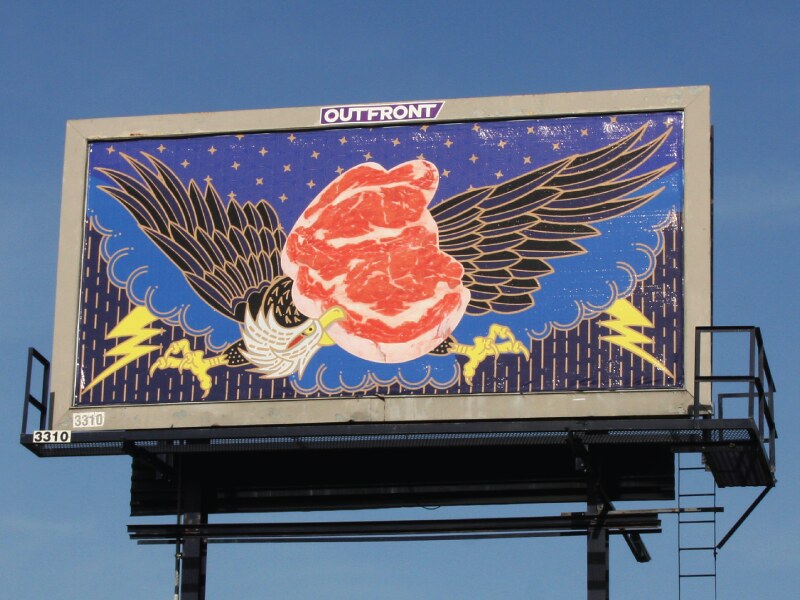A detailed caption for the image could be:

"This striking billboard is supported by two vertical metal beams anchored to the ground, extending upward to a horizontal crossbeam that stabilizes the structure. A sturdy base secures the billboard, while a caged landing area is situated on the right. Adjacent to this on the left is a thin metal ladder providing access to the sign. The billboard itself is framed in gray, crowned at the top with the brand name 'OUTFRONT' in bold white letters, displayed as a single word. Dominating the center of the billboard is a powerful image of an eagle. The eagle spreads its majestic wings wide on either side of a central stake, with its head bent down, gripping the stake firmly in its powerful beak. Its talons are extended, poised as if capturing prey. The background features a vibrant blue sky adorned with stars, adding a patriotic flair. On both the bottom left and right corners of the billboard, dynamic lines and lightning bolts symbolize rain and thunderstorms, adding an element of dramatic tension to the overall composition."